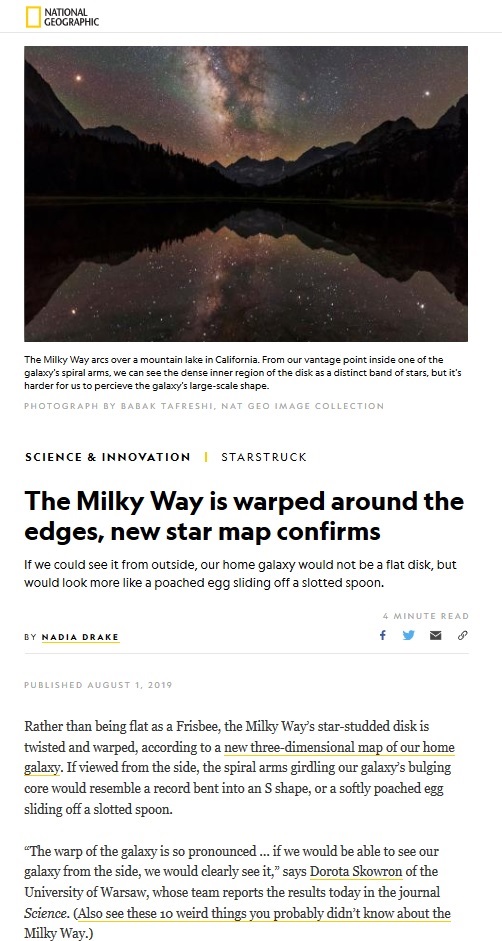**National Geographic**

In the upper left corner, a small yellow square is positioned beside the iconic "National Geographic" text. Below, a captivating image showcases a dark, night sky. At the center, a reddish-white glow peers through dark gray clouds, accompanied by bright red stars flanking the left and right sides of the sky. Towering black mountain peaks dominate the lower portion of the image, reflected in the tranquil waters below, where the stars also glisten.

Descending from the image, the text "Science and Innovation" in all capitals precedes a horizontal line, leading to the word "Starstruck." In bold black text, the caption reads, "The Milky Way is warped around the edges: New star map confirms." A deeper explanation follows, stating, "If we could see it from outside, our home galaxy would not be a flat disk, but would look more like a poached egg sliding off a slotted spoon." The article is attributed to Medea Deake, with the author's name underlined in light yellow.

Further down, two paragraphs are inscribed, with the first highlighting a key sentence underlined in yellow: "A new three-dimensional map of our home galaxy." The second paragraph, also underlined in yellow and enclosed in parentheses, suggests additional reading: "Also see these so weird things you probably didn't know about the Milky Way."